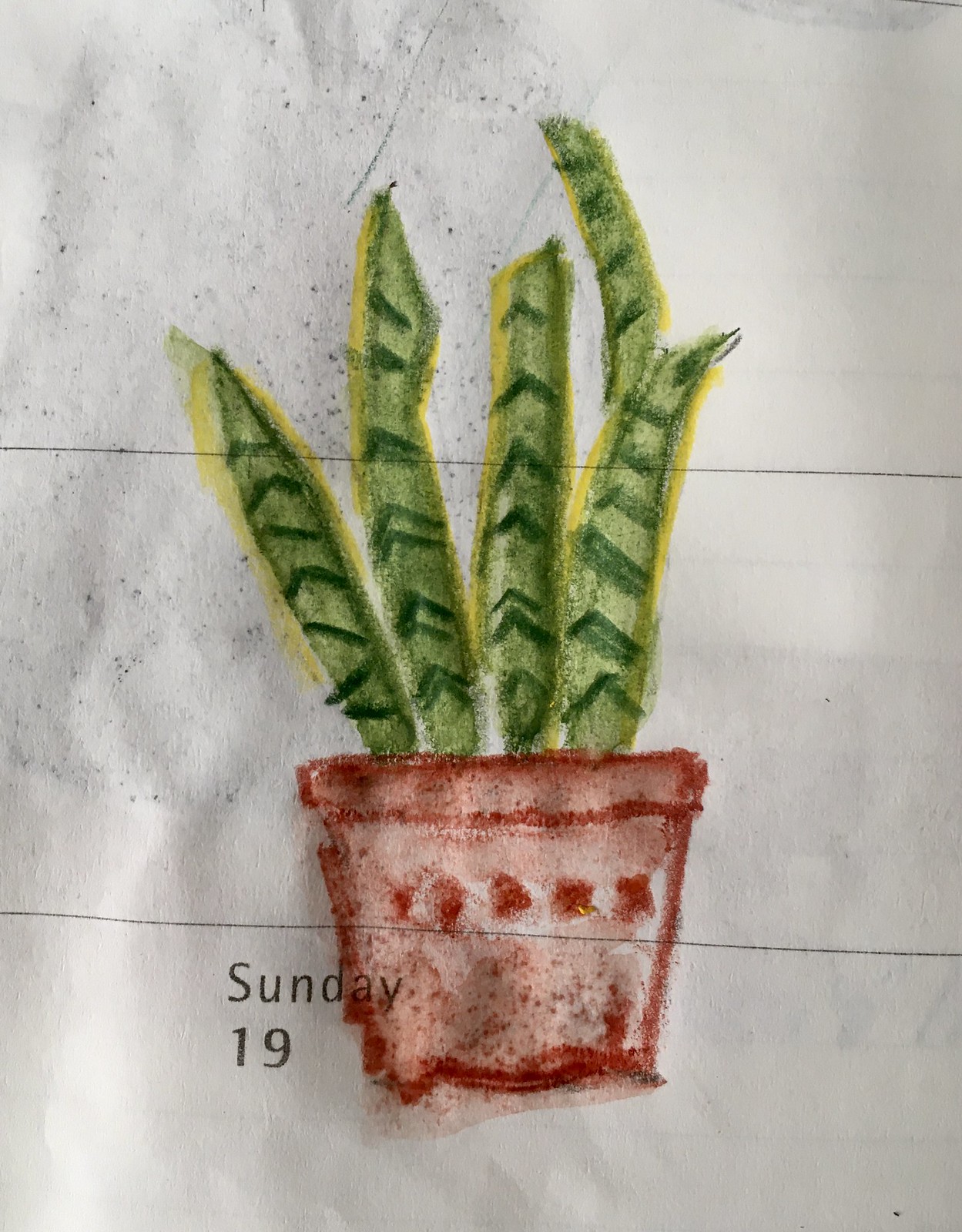The image is a photograph of a child's drawing on a piece of paper divided by two horizontal lines, slightly tipped downward on the right. The drawing depicts a house plant in a reddish-brown pot with five reddish-brown dots forming a horizontal line near the middle-top of the pot, which is slightly tipped to the left. The plant exhibits four long, skinny green stems or leaves, with the one on the right splitting into two nearer the top, making it appear as five stems at the top section. Each leaf is detailed with a dark green line and a yellow outline. The paper appears to be from a calendar, as indicated by the text "Sunday 19" typed in black letters on the bottom left corner, overlapping with the pot. The overall drawing is a mix of light and dark green hues, accented with yellow borders around the leaves, giving the plant a slightly whimsical and delicate look.